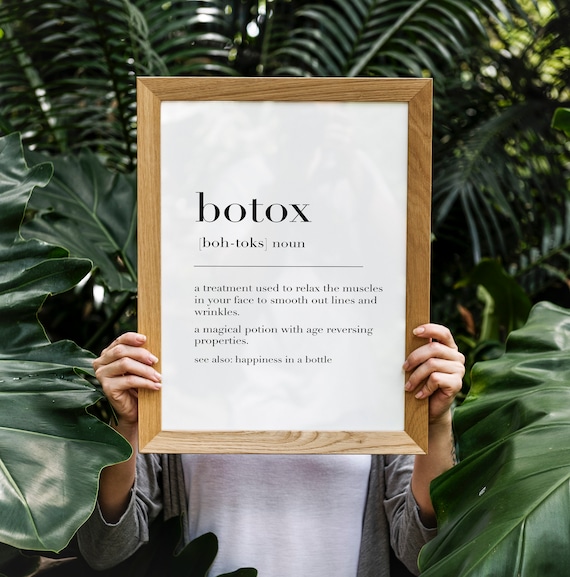In this perfectly square color photograph, a person stands facing the camera, obscured by a large, rectangular wooden frame they are holding up, which covers their face. The background is filled with large, dark green leafy plants, including ferns, palm leaves, and philodendrons, all slightly out of focus to emphasize the subject. The frame has a light to medium brown tone and contains a white piece of paper with black text. The text reads: "Botox. noun: A treatment used to relax the muscles in your face to smooth out lines and wrinkles. A magical potion with age-reversing properties. See also: happiness in a bottle." The person, wearing a white t-shirt and an unbuttoned grayish-tan jacket that reaches their elbows, reveals only their hands, which are grasping either side of the frame. The background's lush greenery contrasts with the simplicity of the white paper and black text, making the message the central focus of the image.